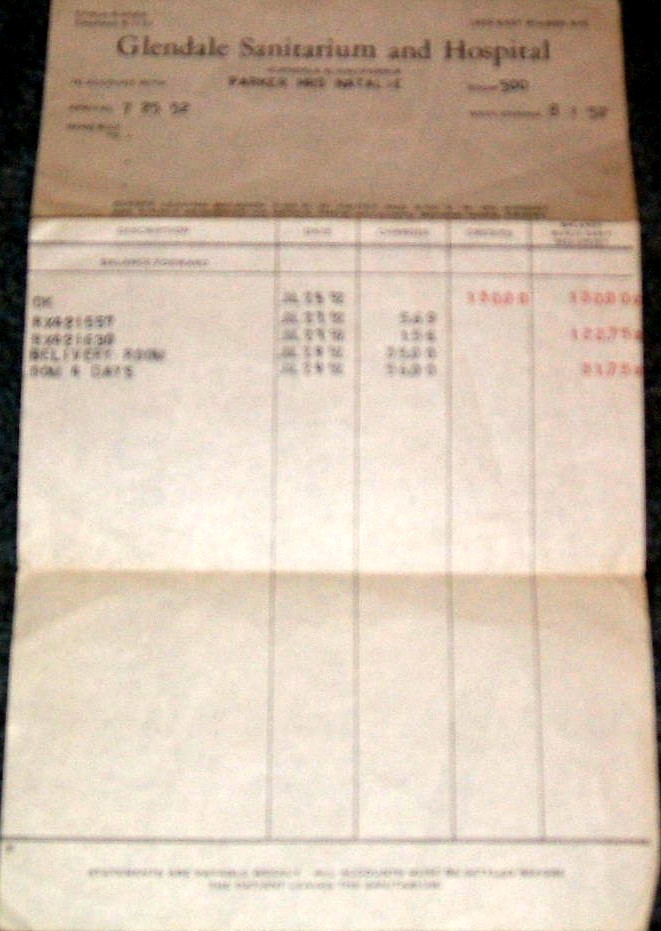This vertical rectangular color snapshot displays a historical hospital bill from Glendale Sanitarium and Hospital, dated from 1958. The bill has been notably aged and folded several times, creating a worn appearance. At the top left corner, although blurry, you can discern the hospital's phone number and address. The prominent text "Glendale Sanitarium and Hospital" stands out in dark brown writing, placed on a light brown section of the paper. Below this header, an itemized list of treatments is provided, though specific details remain illegible due to blurriness. The cream-colored lower portion of the bill features multiple columns: the first few in black print and the last two columns in bright red. Some visible dates suggest services were rendered around July 25th, potentially of 1958. The entire background of the paper is black, enhancing the vintage feel of the document. Despite the worn and blurred text, the layout and scarce numbers evoke an old-fashioned itemized medical statement.